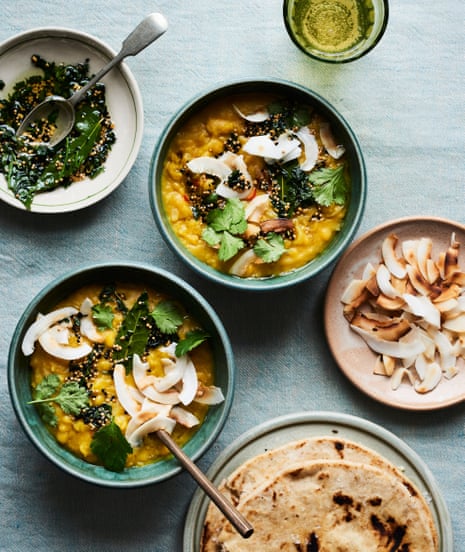A top-down shot of a spread of various dishes arranged on a stone countertop reveals a tantalizing assortment of food, likely with Mexican influences. On the far left, a white bowl containing leafy vegetables dressed in a sauce, with a silver spoon resting in it, could suggest a type of seaweed or herb hot sauce with chili seeds and dark chilies. Moving rightward, a clear glass filled with a yellowish, bubbly beverage, possibly ginger ale, stands out. 

At the center, two matching dark green bowls hold a rich yellow soup, potentially a coconut curry or tortilla soup. The soup is garnished with light-colored, possibly toasted coconut slices or mushrooms, bits of corn, and green leaves, adding to its flavorful profile. Each bowl seems to hold the same dish, though the garnishes differ slightly.

Continuing toward the right, there is a cream-colored bowl with more light-colored slices, possibly mushrooms, adding to the soup's composition. Adjacent to this, a plate holding what could be white chicken or tortilla strips adds a protein element. Lastly, another plate features two stacked pieces of flatbread or charred pita breads. This thoughtfully presented assortment suggests a rich, multi-textured culinary experience with elements of spice, freshness, and warmth.